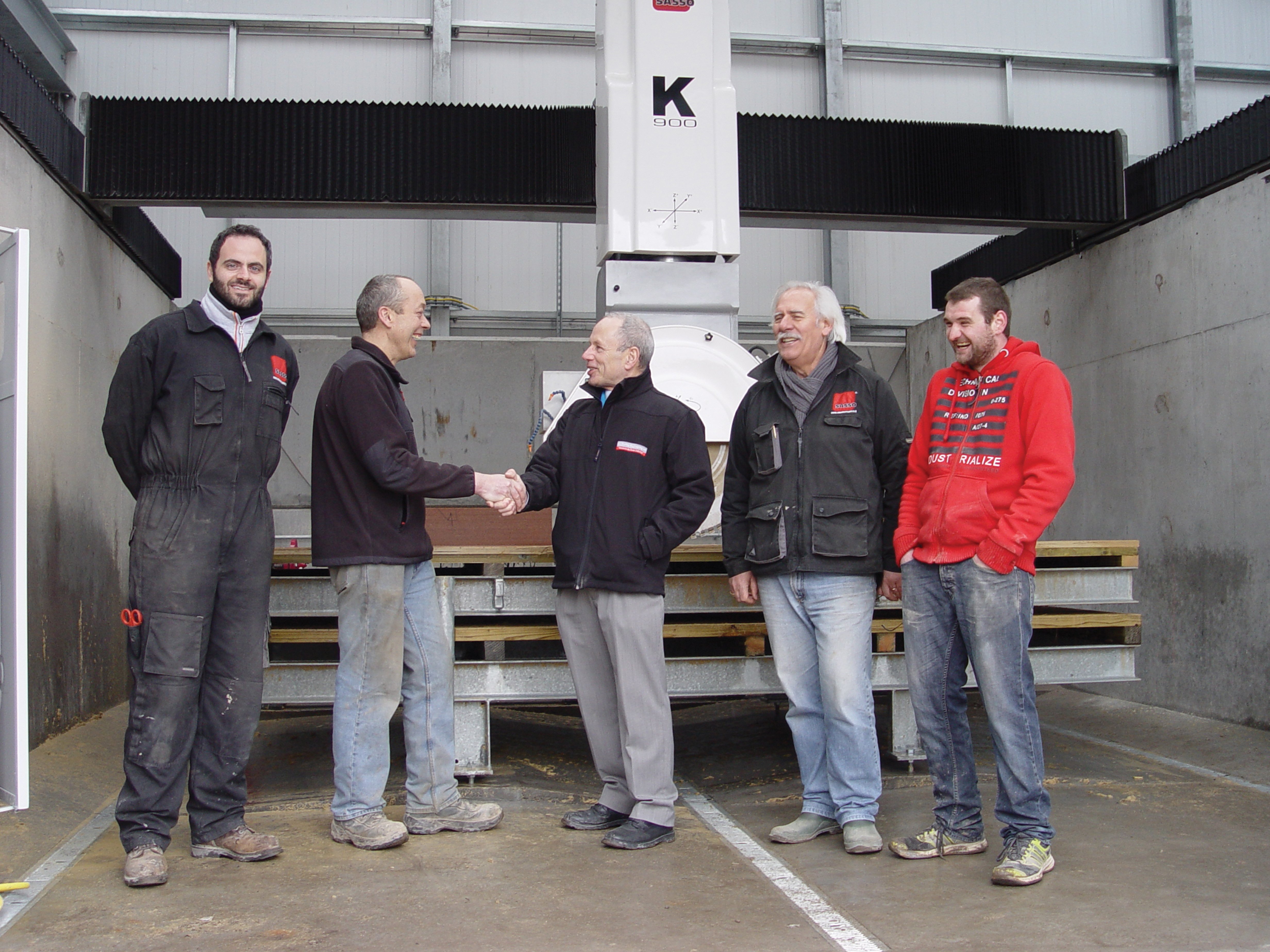The photograph depicts a group of five men standing in a warehouse or factory setting, characterized by grey concrete walls, a silver metal back wall, and a concrete floor marked with white stripes. The background includes large machinery and a pillar marked "K 900," with steel I-beams and wood pallets positioned around. The group is gathered on what seems to be a loading dock, possibly taking a break after a hard day of work, as indicated by their dirty work clothes.

On the far left stands a tall, younger man in his thirties wearing black coveralls with a red logo on the top left shoulder. He has brown boots and a pair of scissors in one of his coverall pockets. Next to him, two men are shaking hands and smiling. One is dressed in a fleece pullover with dirty blue jeans and work boots, while the other, who looks cleaner, wears a black jacket, gray slacks, and black shoes—suggesting he might be a supervisor or owner. Both of these men appear to be in their fifties or sixties.

The fourth man has longish hair and wears a black jacket, blue jeans, grey shoes, and a scarf, seemingly also in his fifties. Finally, on the far right, stands a younger man in his twenties or thirties, dressed in a red hoodie with a design that is partially legible, blue jeans, and tennis shoes. He has his hands in his hoodie pockets. 

The overall scene suggests camaraderie and satisfaction, possibly at the end of a workday, with all of them reflecting the ethos of hard working individuals.